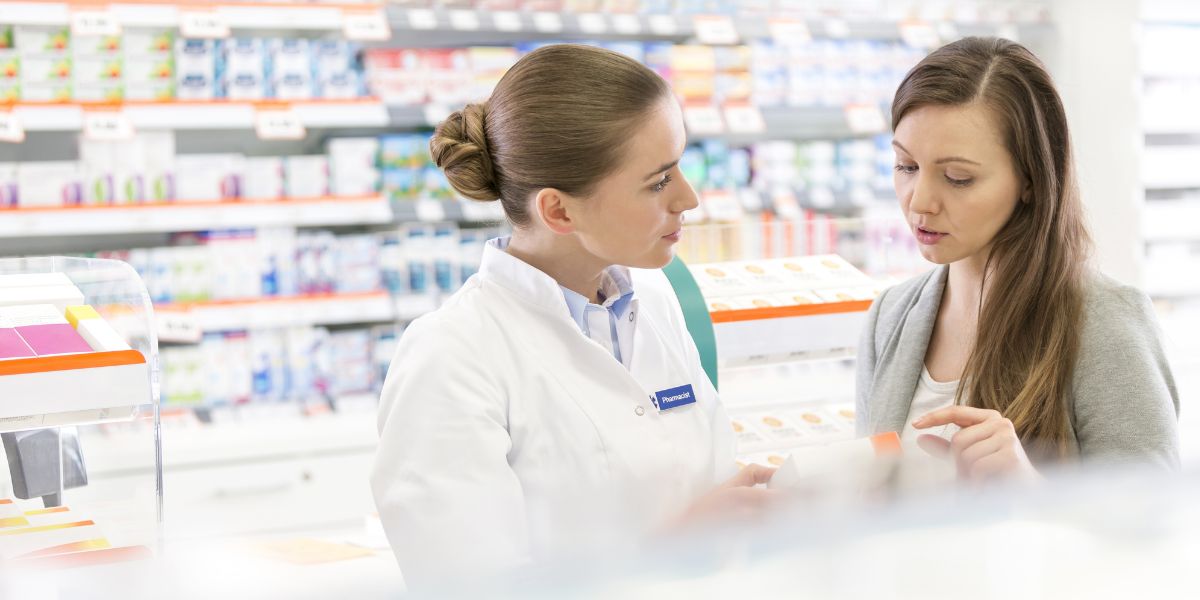In what appears to be a meticulously staged promotional image, a pharmacist and a customer engage in a thoughtful conversation in what looks like a pharmacy section of a store. The scene is sharply defined, with the focus resting primarily on the two women, while the background showcases blurred shelves stocked with boxes of medication that create a professional yet indistinct setting. The pharmacist, easily identifiable by her white lab coat and blue name tag that reads "pharmacist" in white text, has her brown hair neatly tied back in a bun. She stands out, appearing attentive and engaged. The customer, with long, dirty blonde hair draped over one shoulder, is dressed in a gray blazer over a white top. She seems to be explaining something to the pharmacist. The overall polished appearance of the individuals, coupled with the lack of other people and the controlled composition of the scene, underscores the image's promotional intent, ideal for advertising a pharmacy’s customer service.